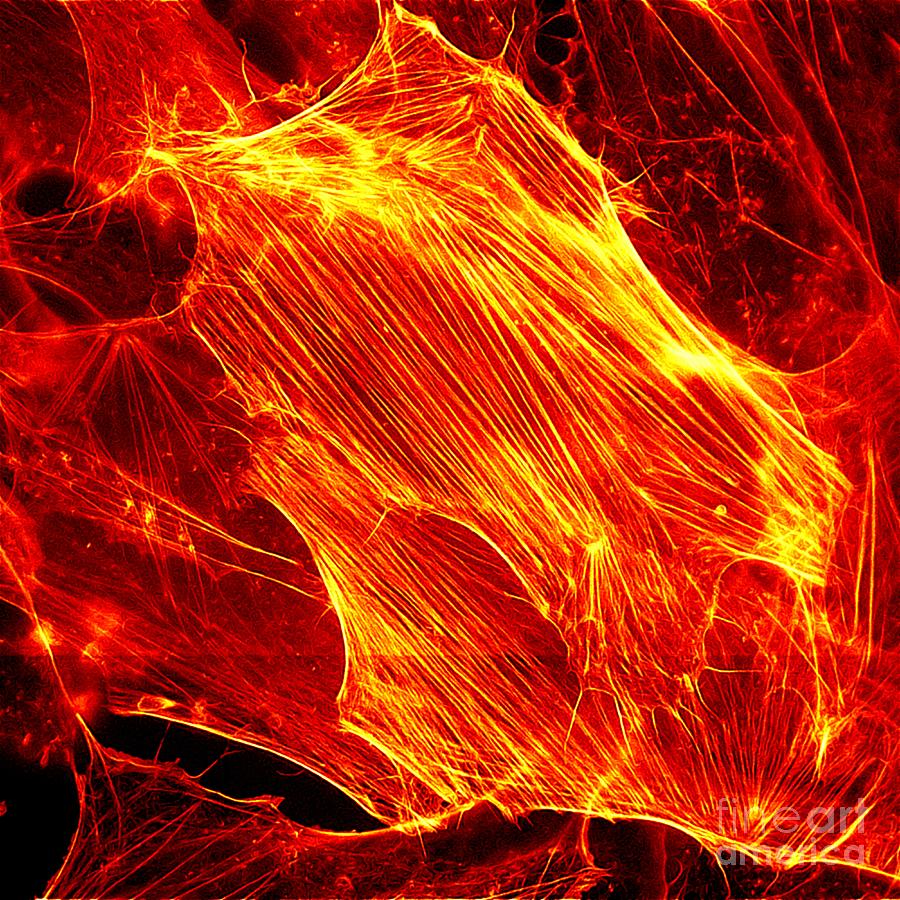The image is a square-shaped light artwork with a black background, featuring vibrant yellow, orange, and red lines forming a complex, web-like pattern that dominates the composition. These lines, which appear to be produced by a moving light captured in a time-lapse photograph, create an intricate design stretching across the image. The upper left section shows a dispersion into smaller clusters and branches, while the lower right displays a dense concentration of these light fibers. The brightly colored lines create a visual effect reminiscent of a spider web set ablaze, with some areas in the corners showing less dense patches. In the lower right corner, there is semi-transparent white text acting as a watermark, reading "fine art" on one line and "America" on the next, all in lowercase letters. The image is somewhat abstract, with certain parts blurring into indistinct, blurry elements that might resemble plants or grass, adding to the intricate and layered visual texture.